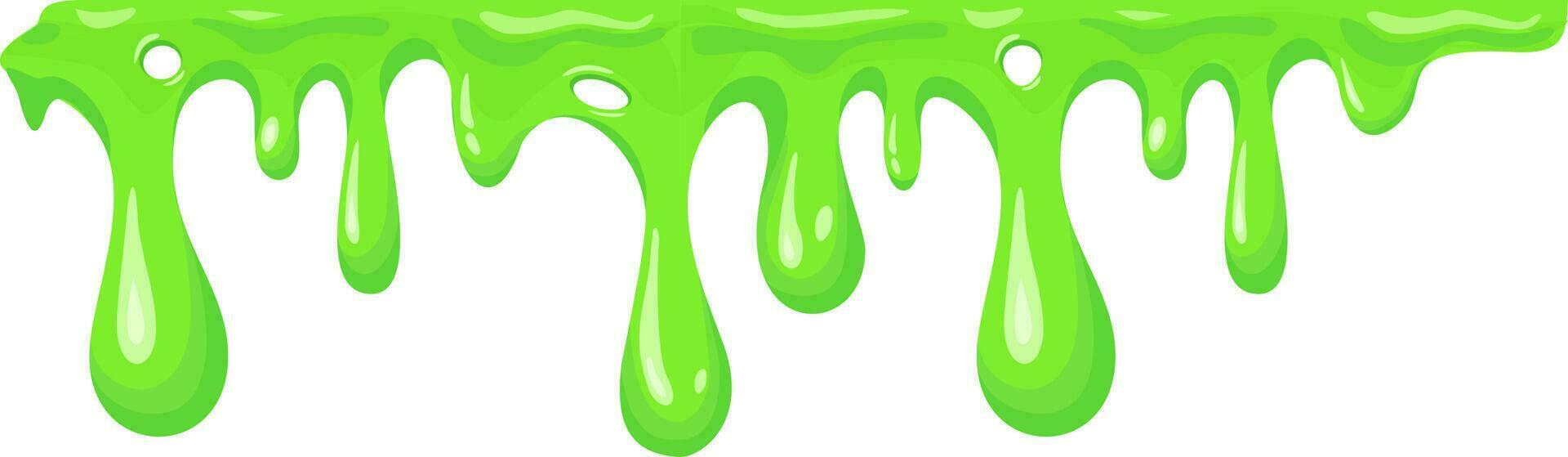This is a graphic, cartoon-style illustration featuring green slime dripping down from a flat ledge against a solid white background. The slime appears in various shades of green, creating a shiny, three-dimensional effect, as if light is reflecting off its surface. The top portion of the illustration is completely covered in green slime, which transitions into multiple drips varying in size, cascading down. The slime also features a few holes, enhancing its gooey, bubbly texture. There are approximately ten to twelve distinct drips depicted in the image. Overall, the illustration combines light and shadow within the slime to accentuate its viscous and glossy appearance.